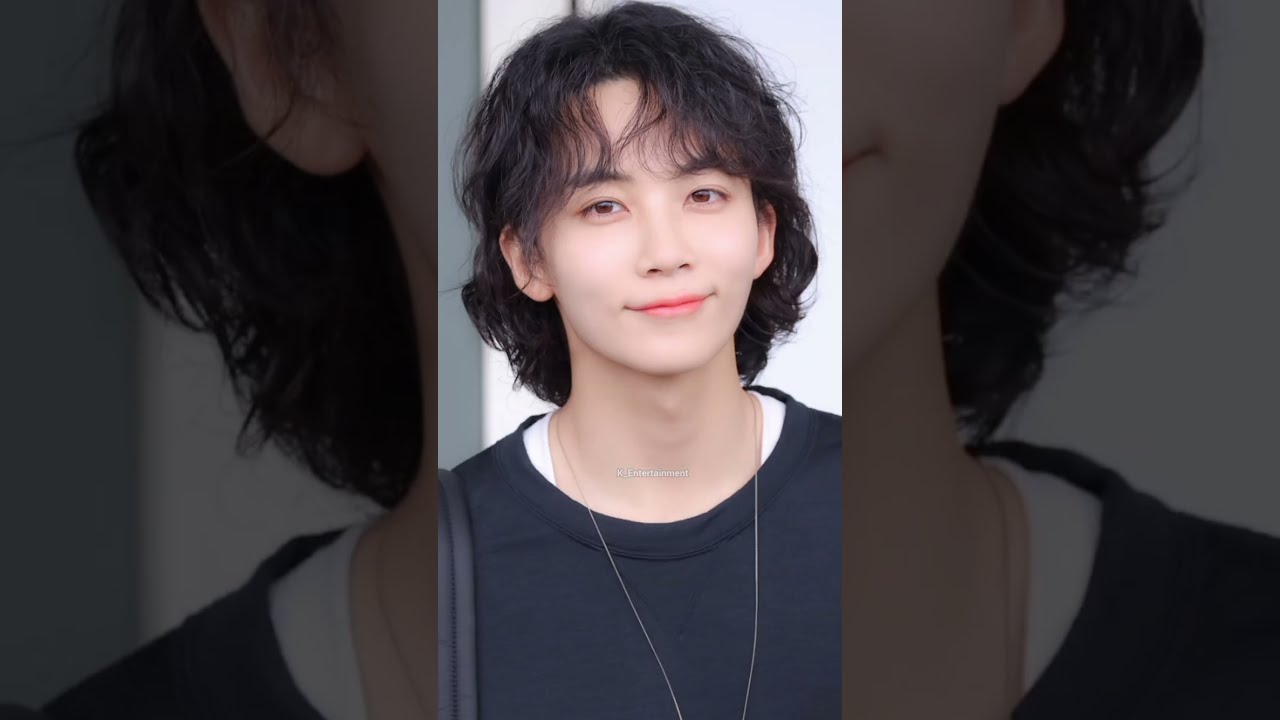The photograph features an Asian man with delicate, feminine features, including dark, shaggy hair that reaches his shoulders and curtain bangs framing his face. His expressive brown eyes and slightly closed-mouth smile enhance his warm and approachable demeanor. The man is adorned with a noticeable long, thin wire necklace that extends beyond the frame of the image. He is dressed in a dark blue, possibly black, sweater over a white undershirt, with the undershirt peeking out at the shoulders. The primary image is centrally located in a vertical rectangle, set against a background that is a darker, enlarged version of the same image, emphasizing the central figure.